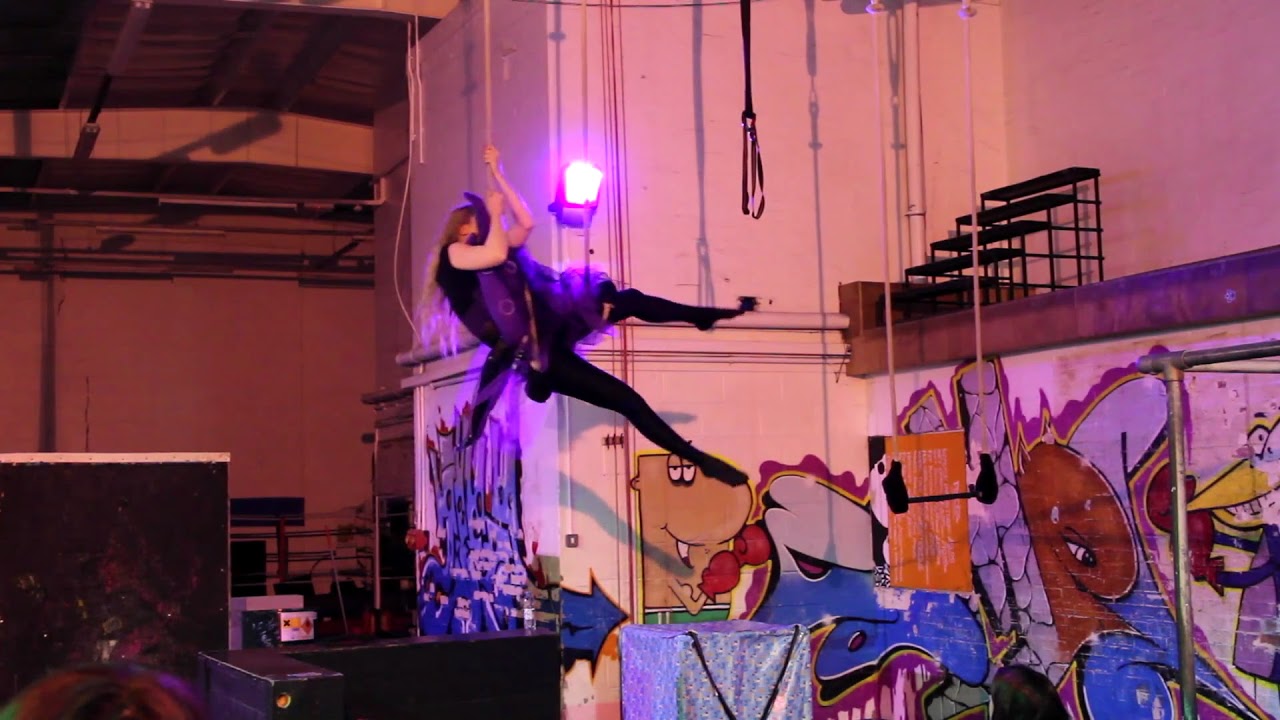In this image, a woman dressed entirely in a black body stocking is the focal point, suspended mid-air as she holds onto a rope hanging from a high ceiling. Her legs are tilted horizontally, showcasing her grace and strength. She has long reddish-blondish hair that adds a striking contrast to her dark outfit. The scene appears to be set in a spacious room with high walls that bear graffiti and abstract paintings, giving off a creative, somewhat chaotic atmosphere. A purple light behind her casts an intriguing shadow, adding to the dramatic effect. Various other ropes hang from the ceiling, suggesting an environment typically found in a gym or theatrical setup. The background reveals a white wall adorned with colorful, cartoonish characters and a large abstract painting, hinting at a whimsical, artistic space. The overall scene exudes a sense of preparation for an aerial performance or gymnastic routine.